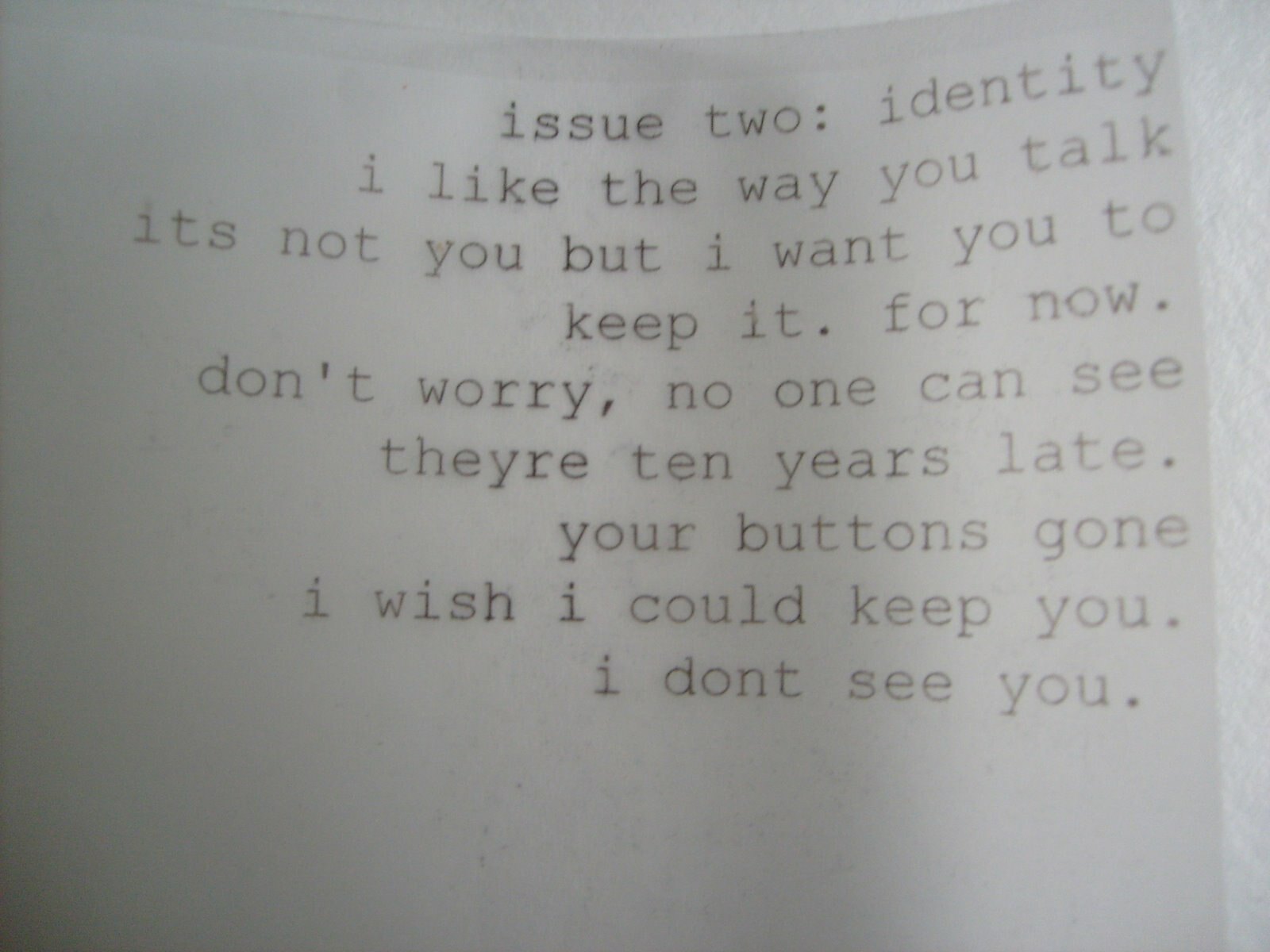The photograph depicts a somewhat worn, white piece of paper with faint black text typed in a consistent Courier-like font, suggestive of a typewriter. The text reads: “issue 2: identity. i like the way you talk. it's not you but i want you to keep it for now. don't worry, no one can see they are 10 years late. your button's gone. i wish i could keep you. i don't see you.” Notably, all the letters are in lowercase. The paper appears slightly bent and curled, particularly on the right side, and seems to be placed on a white, textured surface that resembles a wall. The composition and cryptic nature of the typed message evoke a sense of poetry or a cryptic, emotional note.